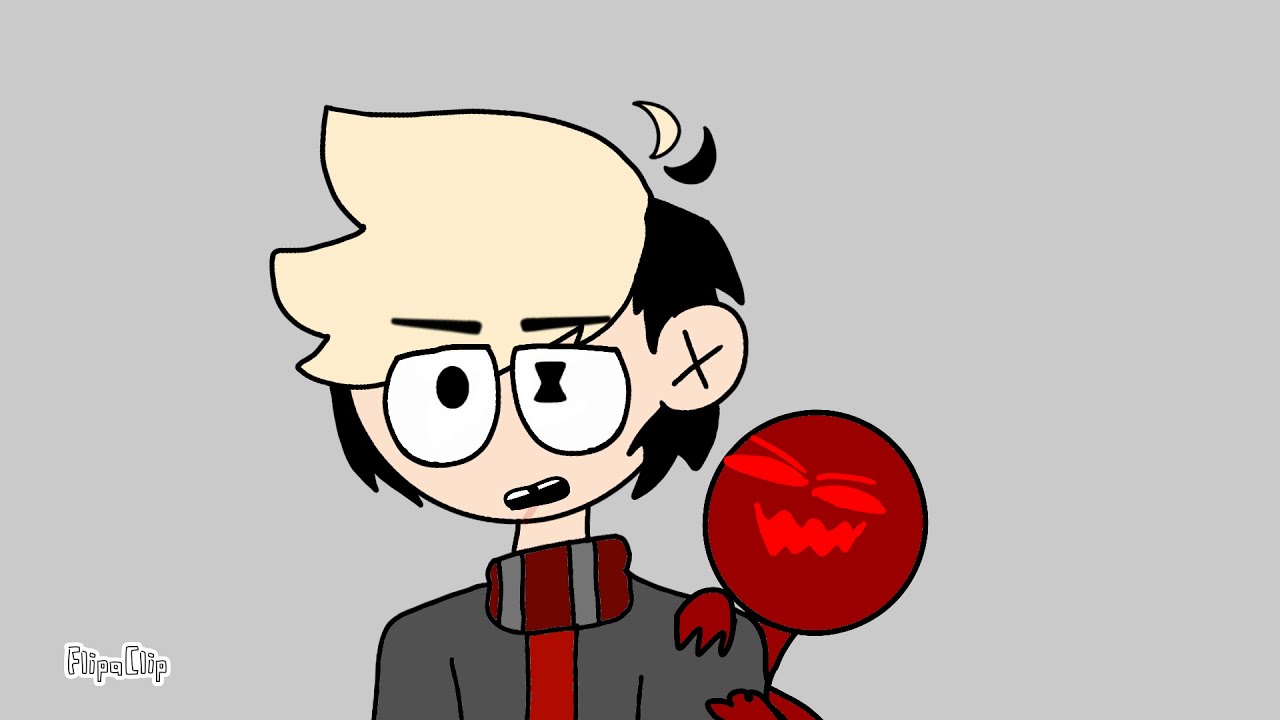A detailed cartoon illustration features a peculiar character with distinctive attributes set against a flat gray background. The central figure sports eyeglasses and exhibits contrasting hair colors: blonde on the top and black at the back. His facial expression is somewhat foolish, with large eyes—one round and the other hourglass-shaped—and a small mouth with gapped teeth. One ear is adorned with a large X mark, adding to his quirky appearance. He is dressed in a gray turtleneck, with a red shirt peeking through and a burgundy and gray scarf draped around his neck. Perched on his left shoulder is a mischievous, devil-like figure with a circular head and jagged teeth, resembling a sinister balloon. The bottom left corner of the image bears the text "FLIPA CLIP" in a cartoonish font, indicating the creator's signature.